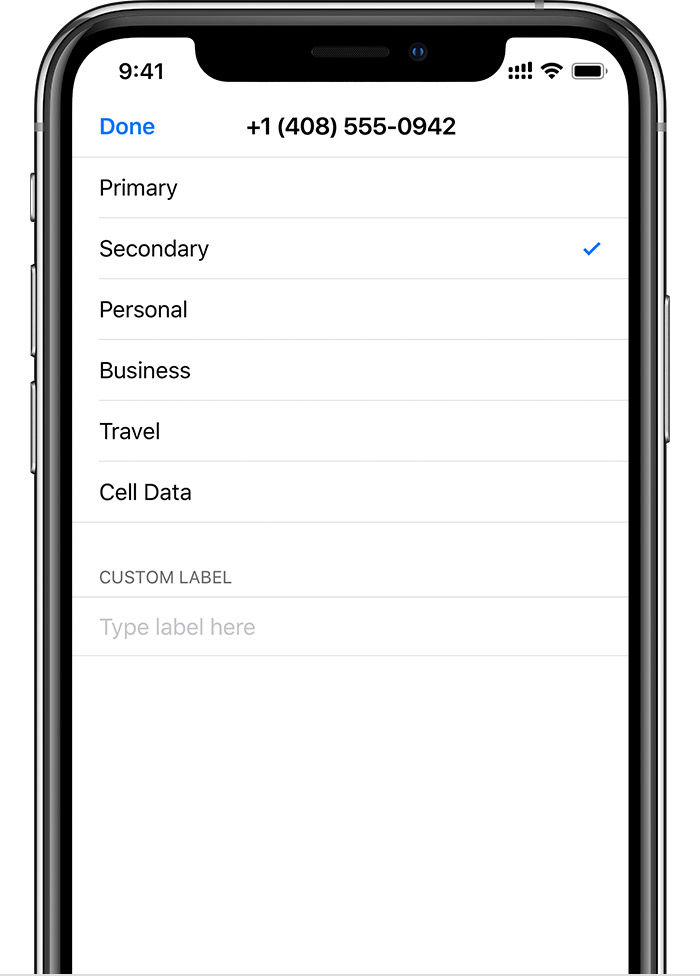This image is a close-up view of a settings screen on a cell phone, showing the outline and physical features of the device itself. The phone appears to have a black body. In the top-left corner of the screen, the time is displayed as 9:41, while in the top-right corner, four signal bars of varying heights indicate cell service strength. Icon indicators show that Bluetooth is enabled and the battery is fully charged. 

At the top of the screen, the word "Done" is highlighted in blue. Below it is a phone number formatted as "+1 (408) 555-0942." The next line down is labeled "Primary," followed by "Secondary" with a check mark on its right side, indicating it is selected. Below these are additional options labeled "Personal," "Business," "Travel," and "Sell Data." At the bottom, an area labeled "Custom Label" features a text box with placeholder text that reads "Type label here." 

The visual elements and the font used suggest that this device is an iPhone. The image also shows the phone's physical buttons, including the mute switch and two volume buttons on the left-hand side, as well as the power button on the right side.